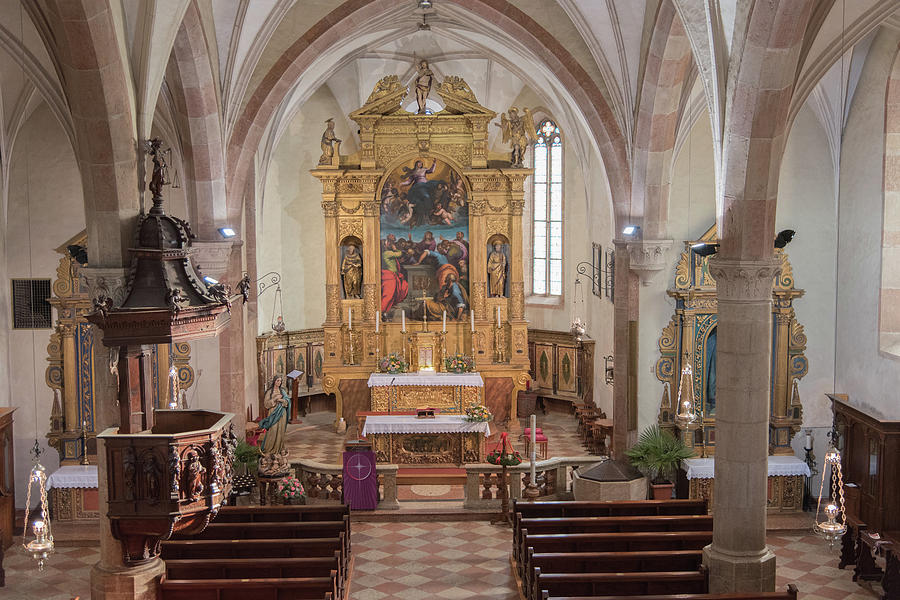The photograph showcases the grand interior of an old, stone-built cathedral, taken from an upper level looking down. Dominating the center is a large, ornately decorated golden altar that stretches from the floor to the ceiling. This altar features a hand-painted depiction of angels and a group of people, possibly including the head of Jesus. Flanking this central image are two recessed windows, each housing statues of saints. Below, a table draped with a white tablecloth displays four candelabras and a central cross. The church has a domed ceiling supported by light brown stone pillars, and the floor is lined with dark wooden pews arranged in rows on either side of the aisle. Shiny furniture and detailed stone arches enhance the historical and reverent atmosphere of the space.